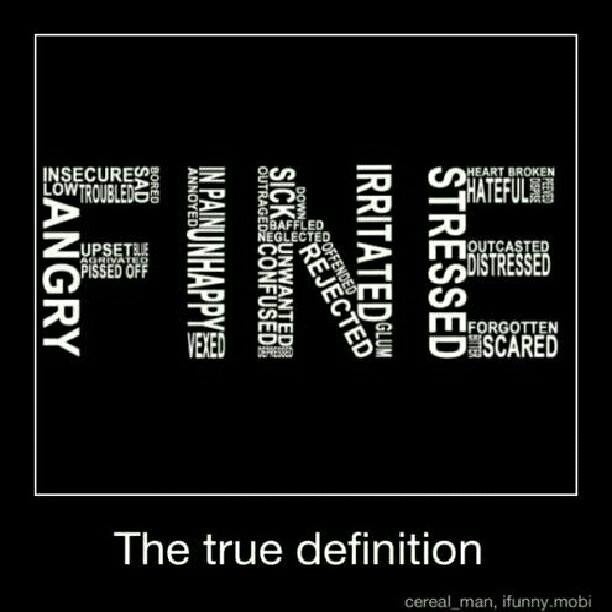The image is a low-resolution digital photograph with a black background and white text. It features the word "FINE" prominently in the center, with each letter of "FINE" constructed from an array of smaller, negative words arranged both horizontally and vertically, in varying font sizes. These words include "insecure," "sad," "bored," "low," "troubled," "angry," "upset," "pissed off," "in pain," "unhappy," "vexed," "annoyed," "sick," "rejected," "offended," "unwanted," "confused," "stressed," "outcasted," and "distressed." These smaller words form the larger letters F, I, N, and E within a white-outlined square that occupies the top two-thirds of the image. Beneath this square, in white text, it reads "the true definition," and in the bottom right corner is a watermark: "serial_man.ifunny.mobi."